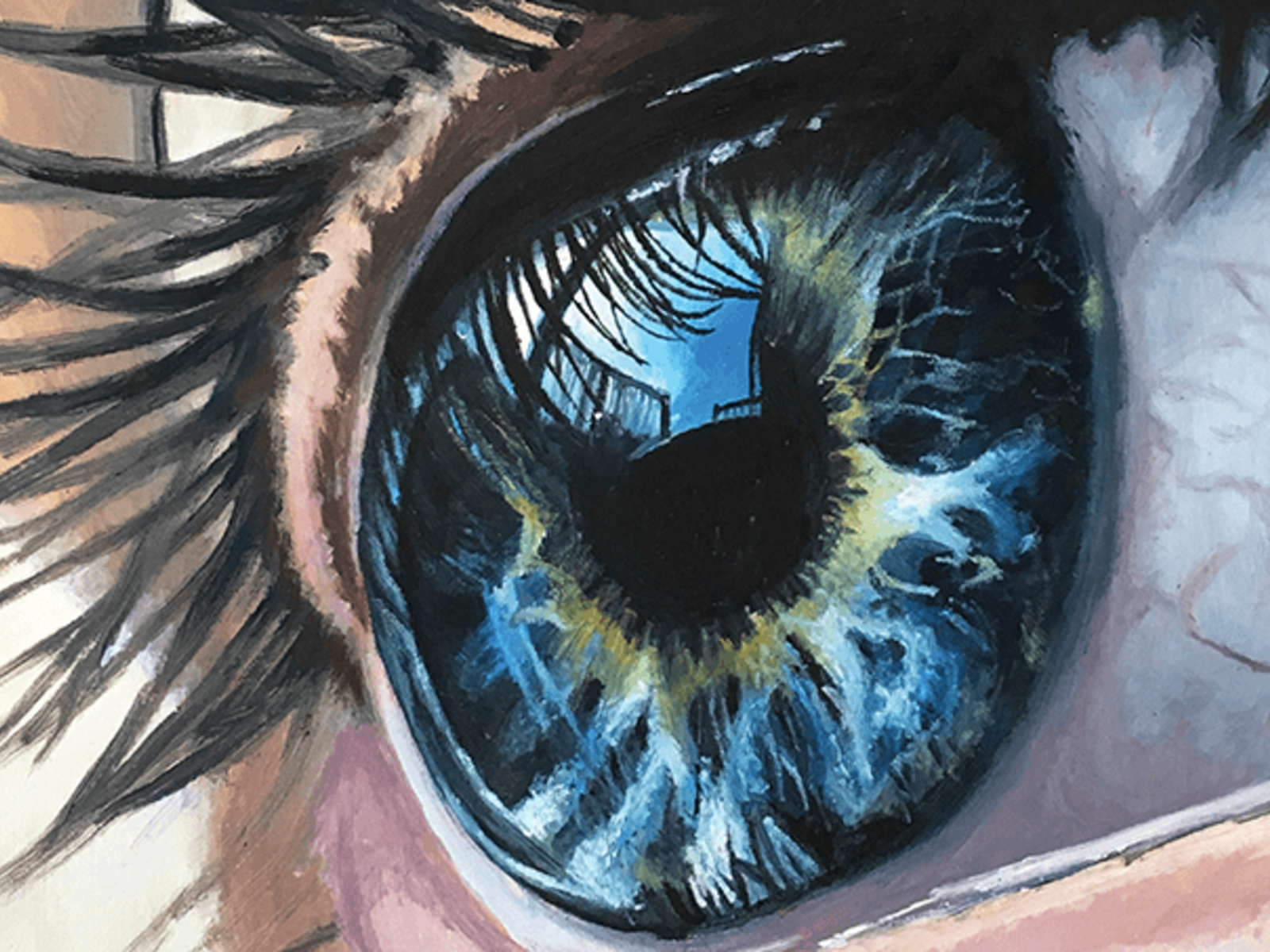The painting is a detailed close-up of an eye, likely created with oil or acrylic paints. The iris, predominantly dark blue with subtle shades of green and yellow, reveals a reflection that suggests the eye is looking at some sort of fencing. The sclera, or the white of the eye, is partially visible, adding to the intricate detail. The upper left part of the painting depicts thick, black eyelashes extending to the left, emphasizing the eye's sideways orientation, as if the subject is lying down. The skin around the eye is captured in light peachy tones, with hints of a dark brown lash line. Below the eye, abstract swirls of pink and white add a touch of surrealism. The entire depiction—including the reflection in the pupil and iris—imbues the painting with a mix of realism and abstraction, leaving an impression of capturing an enigmatic scene within the eye.